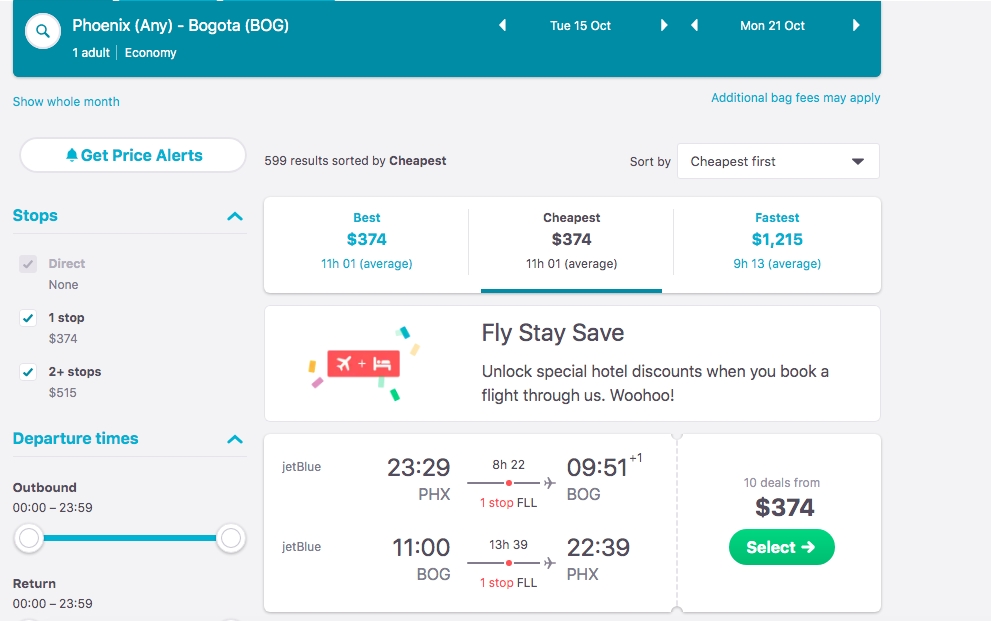A detailed webpage interface is displayed for booking a flight, aimed at users planning to travel from Phoenix to Bogota. The main section of the webpage features a blue box with white text detailing the flight information: "Any flight from Phoenix to Bogota," specifying one adult traveling in economy class. Adjacent to this, a filter option allows users to select travel dates, in this case, Tuesday, October 15th through Monday, October 21st.

Below the flight details, the options "Show whole month" is highlighted in blue text. On the far right, there's a note indicating that "additional bag fees may apply," with a clickable hyperlink for more information on baggage fees.

Further down, there is an option to set up price alerts and to refine search criteria using checkmark boxes, with options for one-stop and two-stop flights currently selected. Users can also specify their preferred departure time, ranging from 00:00 to 23:59 hours.

To the right, a large white box presents various travel options categorized as "Best," "Cheapest," and "Fastest." The "Best" option, highlighted in blue, costs $374 and has a total travel time of 11 hours. The "Cheapest" option also costs $374. The "Fastest" option, priced at $1,215, reduces the travel time to 9 hours. These options include details on the airline, JetBlue, and the respective travel durations.

Finally, a prominent green button encourages users to explore more deals.